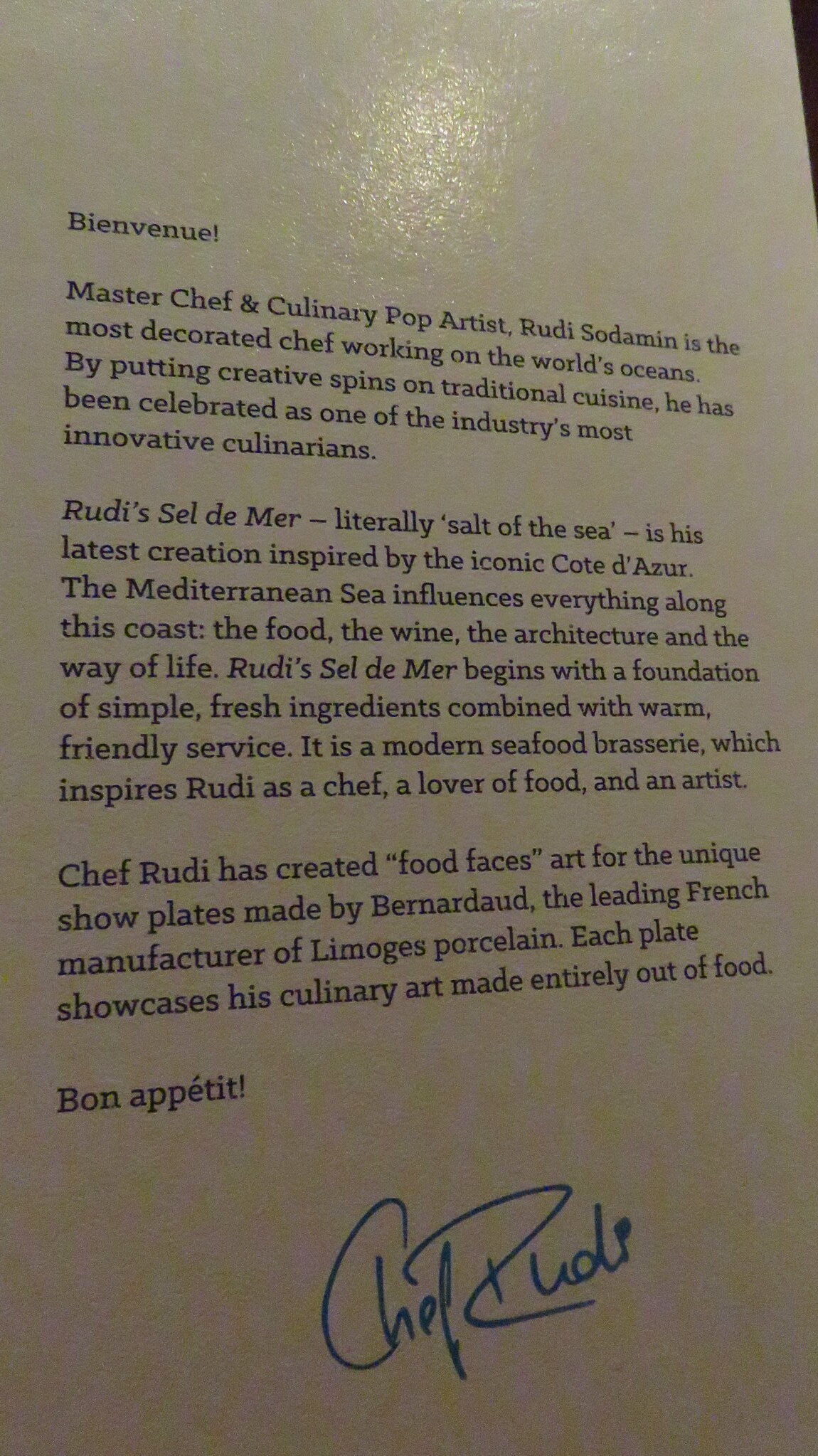The image depicts a glossy white poster board with a printed letter, written in black ink, titled "Bienvenue". The letter highlights Master Chef and culinary pop artist Rudy Sodamin, celebrated as the most decorated chef on the world's oceans for his innovative spins on traditional cuisine. Describing his latest creation, Rudy's Sel de Mer (Salt of the Sea), the letter notes that it draws inspiration from the iconic Côte d'Azur. The Mediterranean Sea profoundly influences the local cuisine, wine, architecture, and lifestyle. Rudy's Sel de Mer features simple, fresh ingredients paired with warm, friendly service, embodying a modern seafood brasserie. Additionally, Chef Rudy's artistic culinary expressions can be seen in his "food faces" art on show plates crafted by Bernard Nod, a leading French manufacturer of Limoges porcelain. The letter concludes with "Bon Appetit" and is signed by Chef Rudy in blue ink.